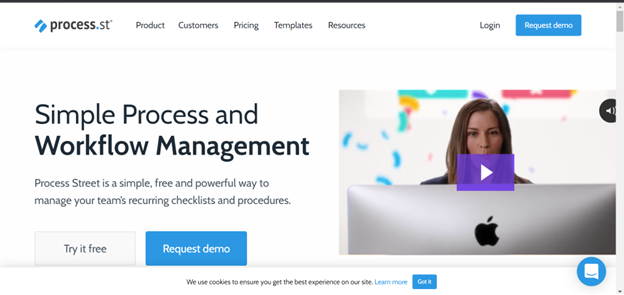This is a detailed caption for the image described:

The image is a screenshot of a website, presented horizontally. The background of the site is white, and the image has a thin black line serving as a border at the top. On the right-hand side, there's a vertical scroll bar. The left side and the bottom do not have visible borders.

At the top of the page, aligned to the left, is a header bar displaying the logo "Process.st." Adjacent to this logo are several categories in small gray text: Product, Customers, Pricing, Templates, and Resources. To the upper right corner of the header, there is a "Login" option and a prominent blue button labeled "Request Demo."

The main content of the webpage is split into two sections. On the left, there is a block of text that reads, "Simple process and workflow management. Process.st is a simple, free, and powerful way to manage your team's recurring checklists and procedures." Beneath this text are two buttons: one labeled "Try it Free" and the other "Request Demo," the latter highlighted with a blue button.

On the right-hand side, there is a photograph featuring a person with their face obscured by a large laptop screen displaying the Apple logo. Superimposed over this person's face is a square translucent purple play button, indicating that it can be pressed to play a demo video.

At the center of the lower edge of the image, there is a disclaimer that reads, "We use cookies to ensure you get the best experience on our site," accompanied by a "Learn more" link and a blue "Got it" button. Additionally, a blue message icon is visible at the lower right-hand corner of the image.